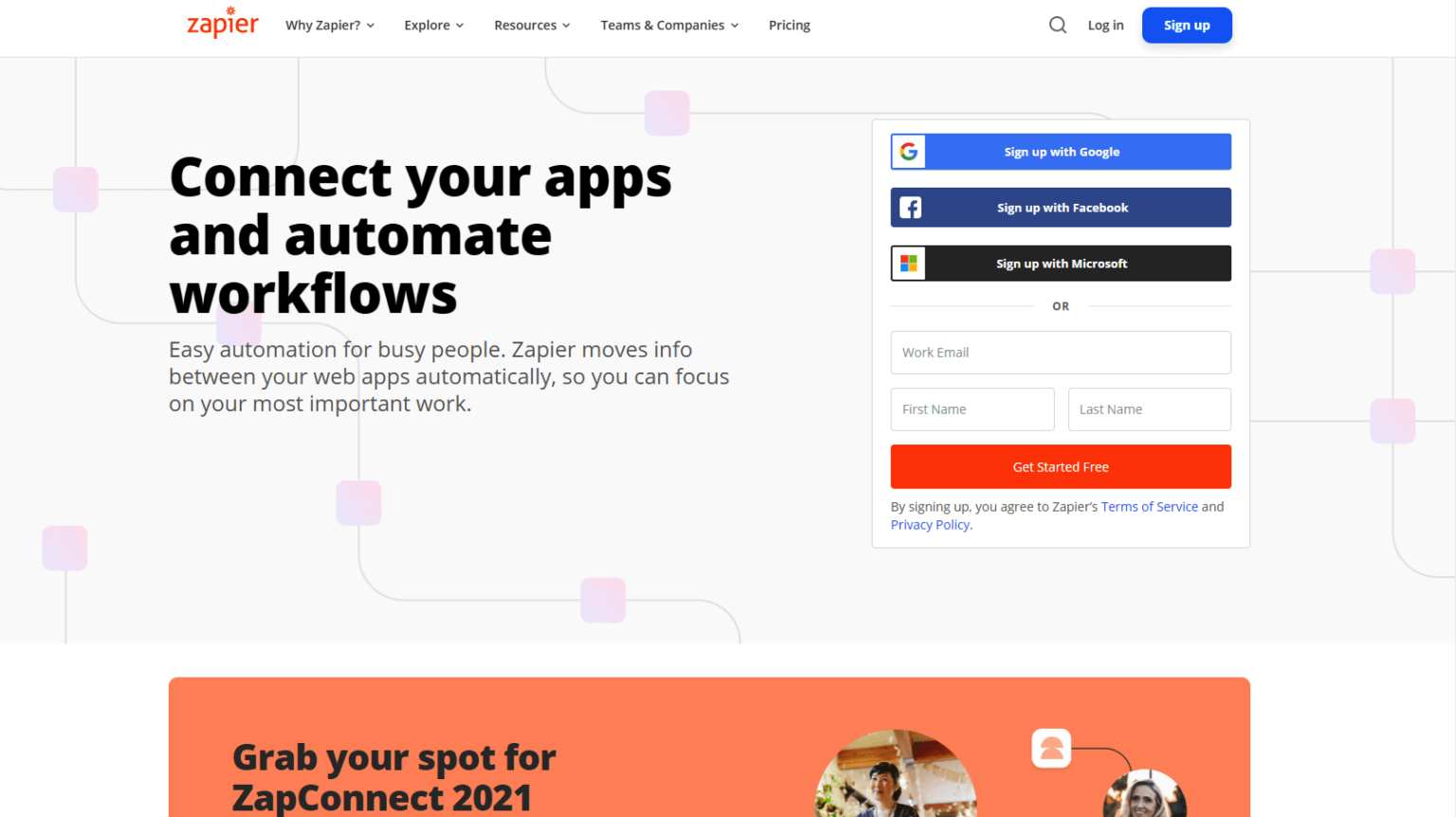This is a web page for the company Zapier, spelled Z-A-P-I-E-R. Located at the top left of the screen is the company logo in orange font. From left to right across the top navigation bar, there are the following hyperlinks each with drop-down menus: "Why Zapier," "Explore," "Resources," and "Teams and Companies," followed by a "Pricing" link. Further to the right, there is a magnifying glass icon for search, a login option, and a sign-up option.

Beneath the sign-up option, there's an interactive box offering multiple sign-up methods: "Sign up with Google," "Sign up with Facebook," "Sign up with Microsoft," or alternatively, fields to enter your work email, first name, and last name manually. Adjacent to these options is an orange button labeled "Get Started Free." Below this button, there's a note indicating that by signing up, users agree to Zapier's terms of service and privacy policy.

Dominating the main body of the web page, prominently displayed on the left, are bold words that read "Connect your apps and automate workflows." In smaller text beneath, it says "Easy automation for busy people. Zapier moves info between your web apps automatically, so you can focus on your most important work."

At the very bottom of the screen, there are images of an Asian woman and a white woman, accompanied by the text "Grab your spot for ZapConnect 2020."